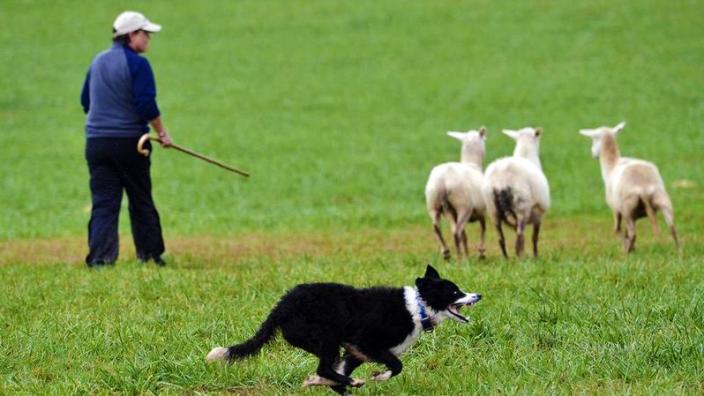In a vibrant green field, a man dressed in black pants, a blue shirt, and a white baseball cap stands to the left of the scene, holding a tan cane in his right hand. His head is turned slightly, revealing the right side of his face. To his right, three white sheep face away from the camera, seemingly moving towards a small hill in the background, where there's nothing but endless grass. In the foreground, a black and white collie runs joyfully from left to right, its mouth open in mid-gallop. The dog's body is predominantly black with a white collar, and its tail is black with a white tip. This outdoor color photograph, taken during the day, captures an action-packed moment in pastoral life.